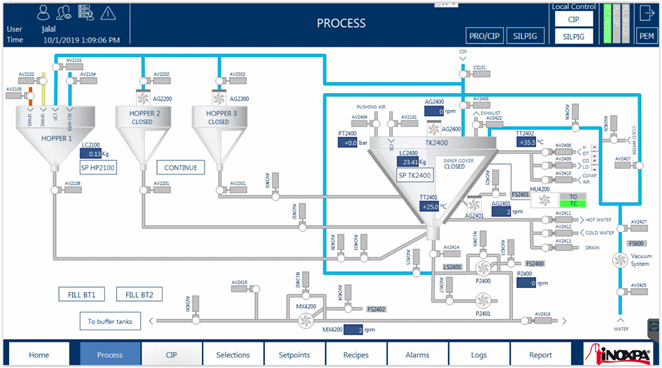The image displays a detailed interface of an automated production system. At the top, a large rectangular blue section features several elements. In the top left, there's an interactable digital user interface labeled "User: Jalal," along with the date "1st October 2019" and the time "1:09 PM." Above Jalal's name, there are four icons depicting a single human, multiple humans, a human with a server, and a caution triangle. A turquoise line separates this section from the rest of the blue area which reads "Process" at its center. To the right are smaller rectangular spaces labeled "Pro/CIP," "SILPIG," and "Load Control," with "CIP" and "SILPIG" beneath it. Adjacent are three vertical spaces: one green and two grey, followed by a turquoise line and a final blue space featuring an arrow pointing right and the text "PEM."

Below this, a large diagram outlines the automated production system. On the left, three hoppers labeled "Hopper 1," "Hopper 2 Closed," and "Hopper 3 Closed" are connected by a production line running horizontally. Various parts of the system are labeled with sequences of letters. A main large triangular hopper icon is centrally placed, with a significant blue line traveling from the left side, across the center, towards this hopper and diverging into other sections.

At the bottom, another user interface in a blue rectangular space includes several white rectangular tabs labeled "Home," "Process," "CIP," "Selections," "Set Points," "Recipes," "Alarms," "Logs," and "Report." The company's logo, "INOXPA," with predominantly red and black text, is situated in the bottom right.